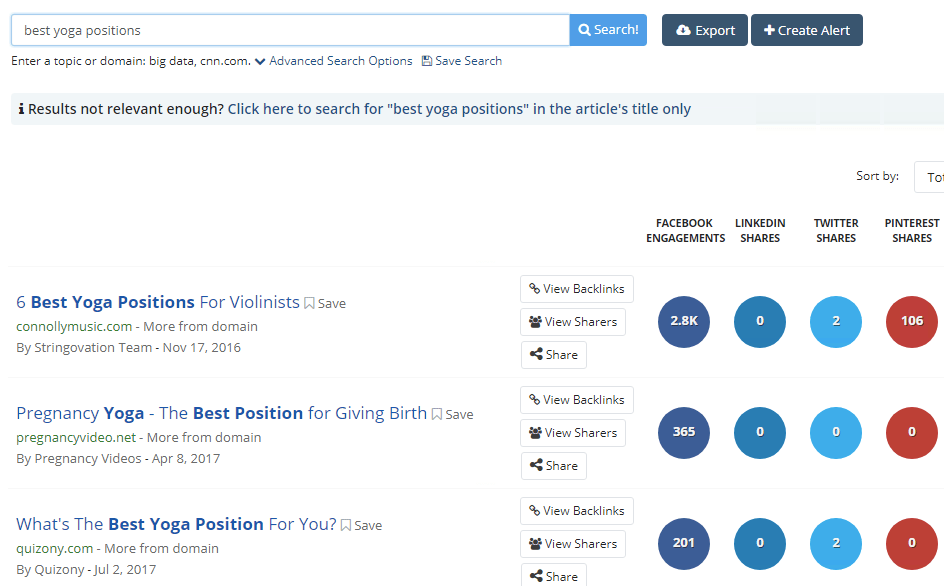This is a screenshot of a web search results page, which doesn't appear to be from Chrome. In the top-left corner, there is a search box outlined in light blue with the query "best yoga positions" typed in black. On the far right side of the interface, options to "Export" and "Create an alert" are visible. Just below these options, there's a prompt stating, "Results not relevant enough? Click here to search for 'best yoga positions' in the article's title only."

The search yields three results:

1. The first result, titled "Six Best Yoga Positions for Violinists," is from connellymusic.com, authored by the StringOvation Team on November 17, 2016. This article has garnered substantial engagement, with 2,800 Facebook engagements, 106 Pinterest shares, but 0 shares on LinkedIn and Twitter. It is notably the most popular link among the three provided.

2. The second result, "Pregnancy Yoga: The Best Position for Giving Birth," is from pregnancyvideo.net, published on April 8, 2017. This article has received 365 Facebook engagements, but no shares on LinkedIn, Twitter, or Pinterest.

3. The third result, "What's the Best Yoga Position for You?" is from quizony.com, dated July 2, 2017. This entry has earned 201 Facebook engagements and 2 Twitter shares, but no shares on LinkedIn or Pinterest.

Each result's popularity and engagement metrics are clearly presented, reflecting user interactions across various social media platforms.